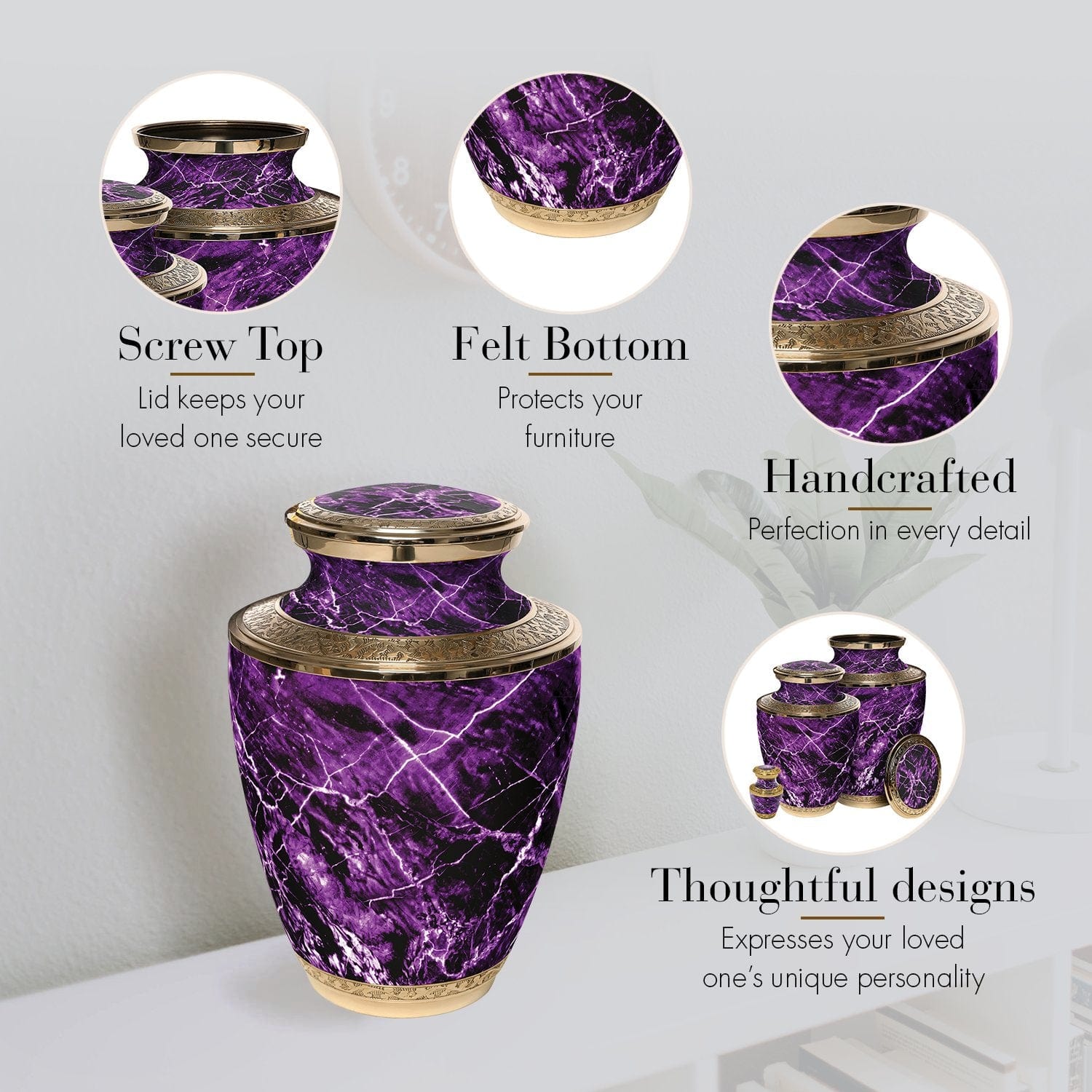This graphic design advertisement showcases an elegantly crafted urn set against a light gray background with an off-white wall. At the center-left, a larger urn is prominently displayed, sitting on a white table near a white cabinet, with a plant in the background to the right. The urn itself is an eye-catching deep purple, with a marbled texture accented by white streaks that resemble lightning, providing a luxurious appearance. It features gold trim at the base and top, highlighting the sophisticated design. 

Above the main urn, there are three smaller circular photographs highlighting different parts of the urn. The captions for these images, all in black text, read: 
1. "Screw top lid keeps your loved one secure."
2. "Felt bottom protects your furniture."
3. "Handcrafted perfection in every detail."

Additionally, in the bottom right corner of the design, there are two images showing a matching set of urns, one larger and one smaller, with the larger urn's lid removed, revealing the same intricate purple marble pattern. Below these images, another caption reads: "Thoughtful designs express your loved one’s unique personality." 

Overall, this advertisement emphasizes the urn's luxurious materials, secure features, and meticulous craftsmanship, providing a fitting tribute to loved ones.